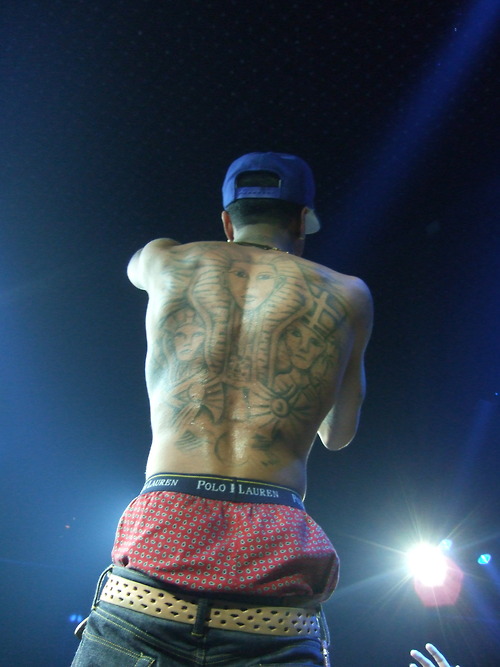In the image, the main focus is a shirtless rapper at a concert, seen from the back. He wears a blue cap and jeans that sag low, revealing his red Polo Lauren boxers with a blue stripe at the top. A tan belt loosely secures his jeans. His back is adorned with extensive tattoos featuring Egyptian themes: a prominent central pharaoh with a headdress that extends from his neck down his spine, flanked by what appears to be Cleopatra on the right and another pharaoh on the left. The tattoos also include elements of sand on his shoulders and possibly a sun and pyramids towards the bottom of his back. The background is dark, likely the stage lighting casting a glow, with a distinct hand reaching up in the lower right corner of the image.